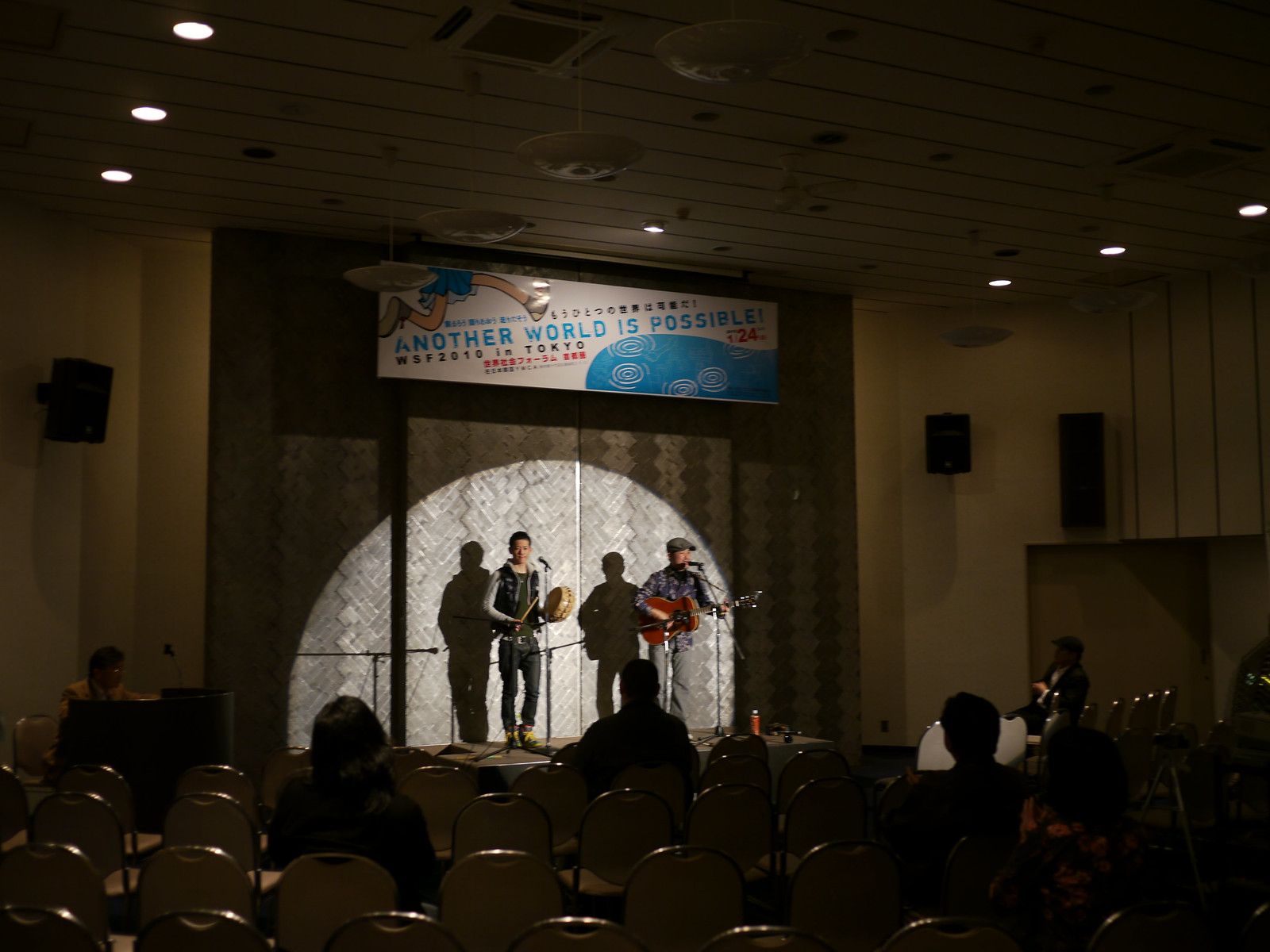This image captures a concert in progress on a dimly lit indoor stage with a sparse audience. At the center of the stage, two men are performing under a spotlight. The man on the right is playing a guitar and positioned in front of a microphone, suggesting he is also singing. On the left, the other man is playing a hand drum, using a drumstick in his right hand and holding the drum with his left. Both performers have their own microphones.

The stage is framed by curtains and lit by overhead lights. There's a backdrop adorned with a large sign that reads "Another World is Possible in Tokyo" in blue letters. The sign also features an illustration of a girl in a blue dress or skirt running, showing her legs and shoes. Additional imagery on the poster includes cartoon-like legs in shorts and sneakers, and a blue drawing with white swirls, possibly representing water.

The photograph is taken from the stands, revealing many empty chairs and only a handful of spectators. The setup resembles more of a makeshift hotel conference room arrangement rather than a full-fledged concert hall. The ambience is somewhat dark, emphasized by the focused lighting on the performers and the overall color palette of the image, which includes shades of tan, white, gray, light blue, red, black, yellow, and orange.